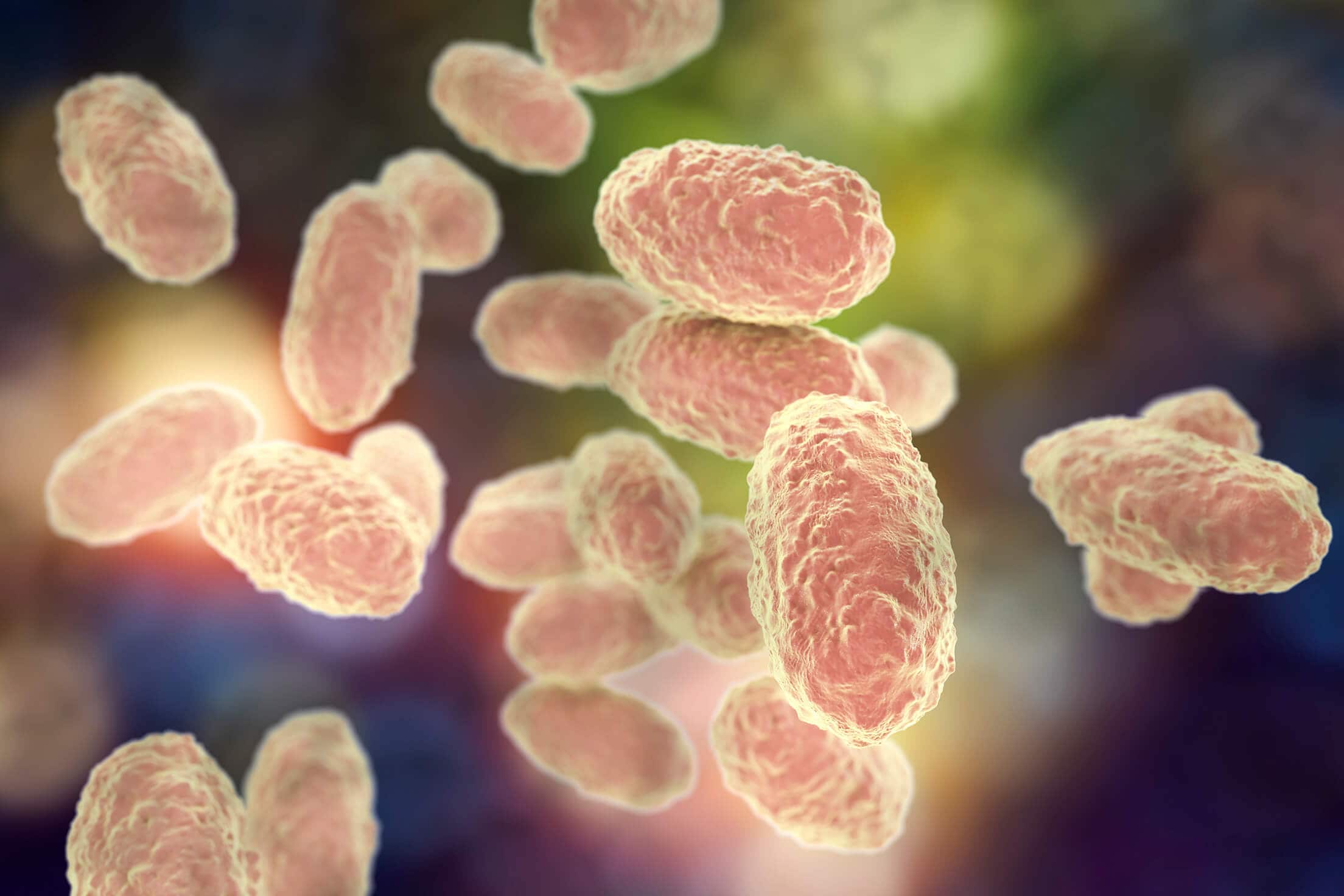A detailed depiction of a landscape-oriented, microscopic slide photo showcases several elliptical, textured shapes resembling cells or bacteria floating in a suspension. These shapes, roughly the size of large pill tablets or grains of rice, have a scaly or bumpy appearance with a red core and a yellowish-beige outer coating that imparts a glowing texture. They are distributed throughout the image, with around 20 prominently in the center, two on the right, and approximately 12 on the left, loosely grouped but not clumped together. The background complements these cells with a mix of blurred light green, almost neon yellowish-green, and dark areas while interspersed with numerous tiny floating particles. This dynamic setting accentuates the vividly colored, suspended bacteria, presumably pertussis bacteria associated with whooping cough, making for a fascinating study of microscopic life forms.